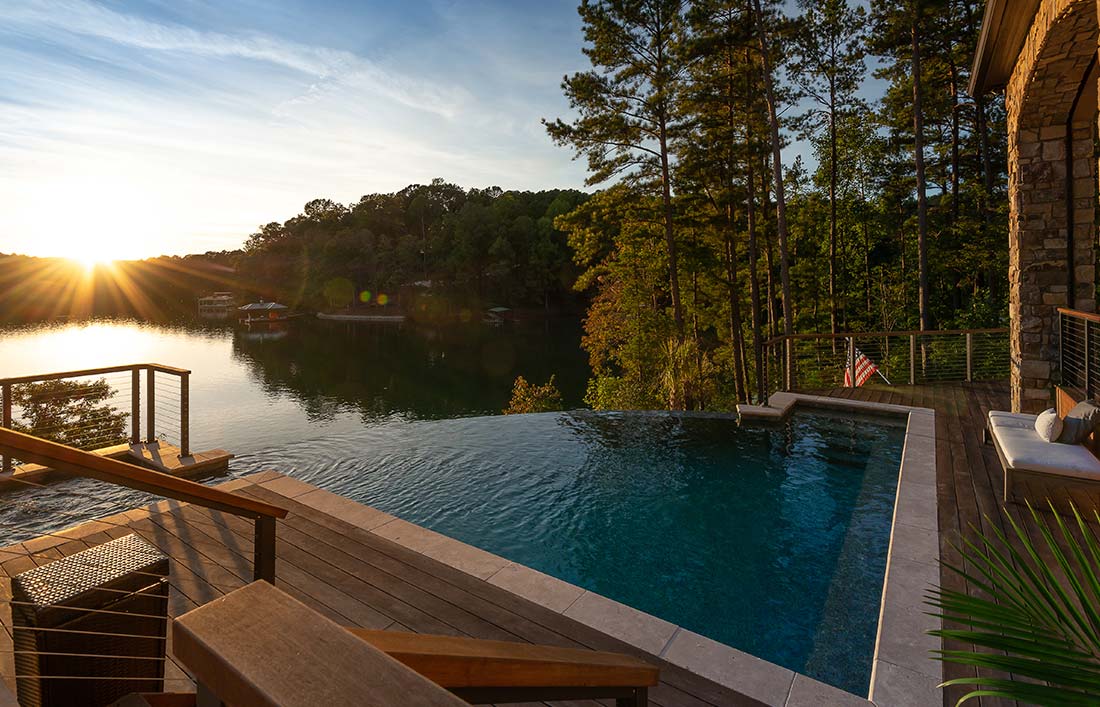This image showcases a modern, scenic outdoor setting featuring a unique pool that creates an optical illusion of blending seamlessly into a lake in the background. The pool, distinctly designed with a triangular shape at the edge and a squared-off rear, is framed by rectangular gray bricks and a wooden dock that surrounds it. The deep blue waters of the pool contrast with the greenish-blue hue of the lake beyond, which is bordered by lush trees and vegetation.

In the center of the image, the pool appears to stretch out towards the lake, giving an illusion of an infinity pool. The sky overhead is a light blue with a few hazy clouds, and the sun is either rising or setting, casting a picturesque glow over the scene. An American flag can be seen in the distance to the right, contributing to the serene and patriotic ambiance.

To the right of the pool is a stone-columned house, and nearby, a bench is situated for relaxation. The patio area features flat stones, stairs with wire railings, and wooden top rails for safety. Overall, the scenic beauty is accentuated by the combination of modern architectural elements and the natural landscape, creating a serene and inviting outdoor retreat.